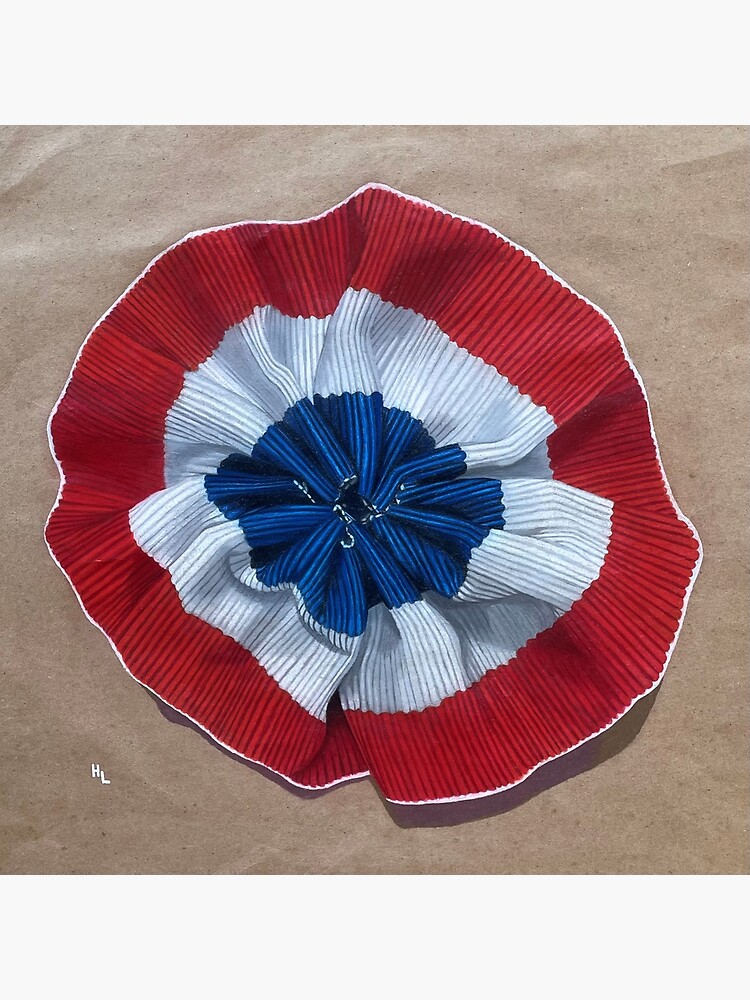The image features a spiral ribbon or circular wrapper, visually akin to a cupcake liner or medal ribbon, intricately ruffled and curled up, giving it a flower-like appearance. The ribbon is composed of three concentric bands of color: the innermost being blue, followed by a white middle ring, and encircled by a red outer band. This colorful object rests on a sandy or beige-textured surface. In the bottom left corner of the image, small bold letters "HL" are subtly inscribed. The whole object roughly spans eight to ten inches in diameter, although the exact nature—whether a hair tie, napkin, or any specific item—remains indeterminate.